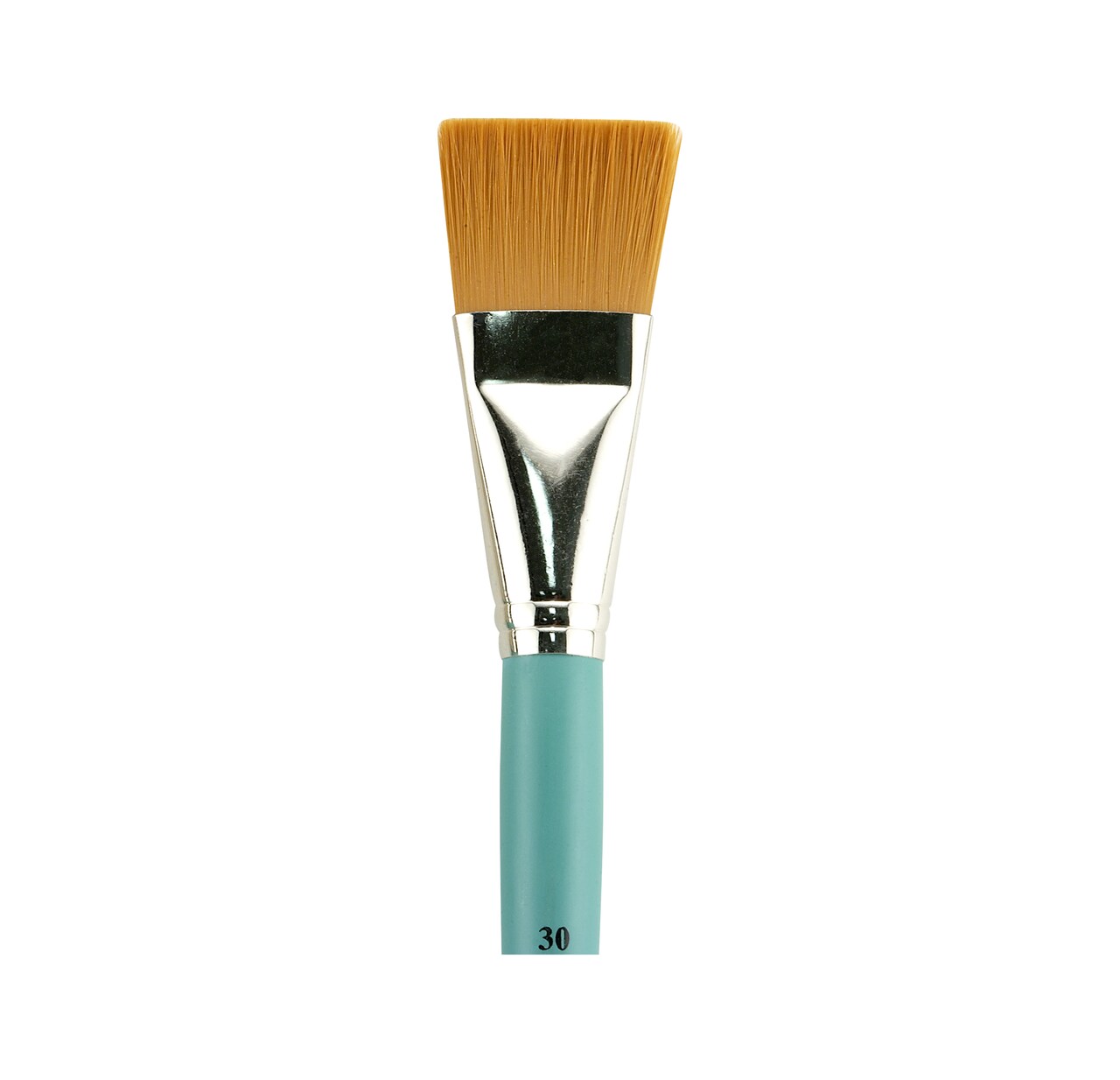This image features a detailed view of a paintbrush against a white background. The brush has a shiny, reflective silver ferrule that securely holds the tightly gathered bristles, which are about an inch long and range from a tan to a dark yellow color. The ferrule is crimped at the top and adorned with two lines at the bottom. Partially visible is the top portion of the handle, which is a vibrant turquoise blue with the number 30 printed in bold black text, indicating the brush size. While the bristles' material is not specified, the brush appears to be a standard utility paintbrush rather than a specialized artistic or makeup brush.